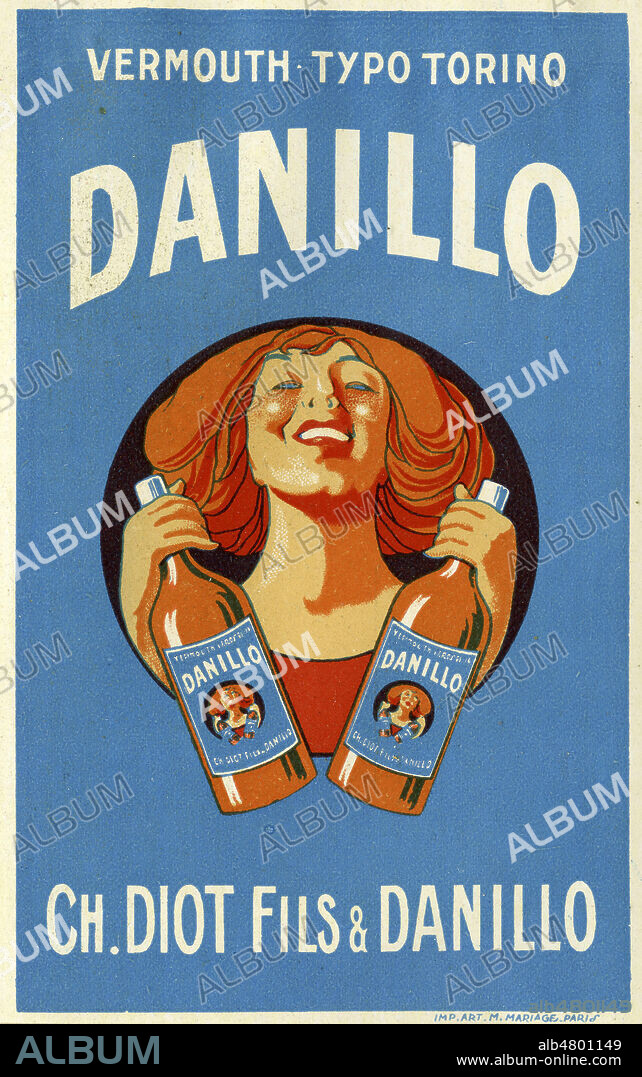The image is an advertisement for an alcoholic drink, specifically vermouth, with the visual style of a drawing or cartoon. The central figure is a smiling, young woman with red hair and red cheeks, dressed in an orange or red shirt. She holds two bottles of a drink called Danilo, each featuring a label depicting her own image. The background of the advertisement is a bright blue, with white text reading "Vermouth, Typo Torino" at the top, followed by "Danilo" in a curved white font. The lower section features a black band with light blue text that reads "album," and the URL www.albumonline.com is also mentioned. Additionally, the words "CH . D I O T Feast Danilo" are written below the woman in white font, and the word "album" is watermarked repeatedly across the image. This eye-catching graphic blends elements of an album cover and a promotional poster.